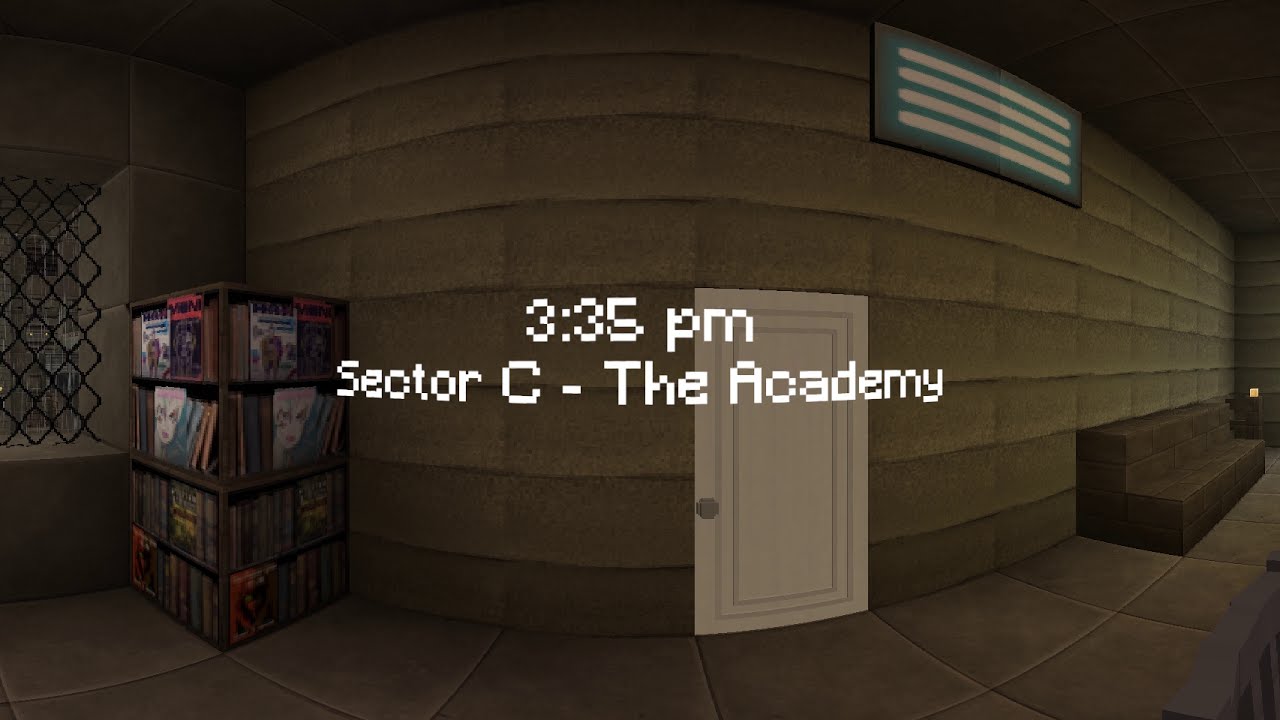The image appears to be a screen capture from a video game, taken indoors in landscape mode, revealing a detailed virtual environment. The scene is set around 3:35 p.m., as indicated by white digital text at the center of the screen, which also denotes the location as "Sector C - The Academy." The room features a brick wall with a white door equipped with a knob situated slightly right of center. The wall bulges outward in the middle, giving it a rounded appearance that tapers off to the sides. Overhead, a rectangular vent with blue outlines and white ovals is positioned on the right side of the wall.

In the lower right corner, concrete blocks form what appears to be either a long couch or steps. Toward the left side, a square, revolving magazine rack or bookshelf occupies the corner, showcasing identical copies of books or magazines on both sides. A solid brown bench is also positioned nearby. The flooring consists of large, brownstone tiles, complementing the rectangular, brown-colored concrete wall.

To the far left of the frame, there is a window with a crisscross grate, contributing a sense of depth and realism to the virtual room. The meticulous attention to detail in the architecture and furnishing suggests an immersive environment within the game.